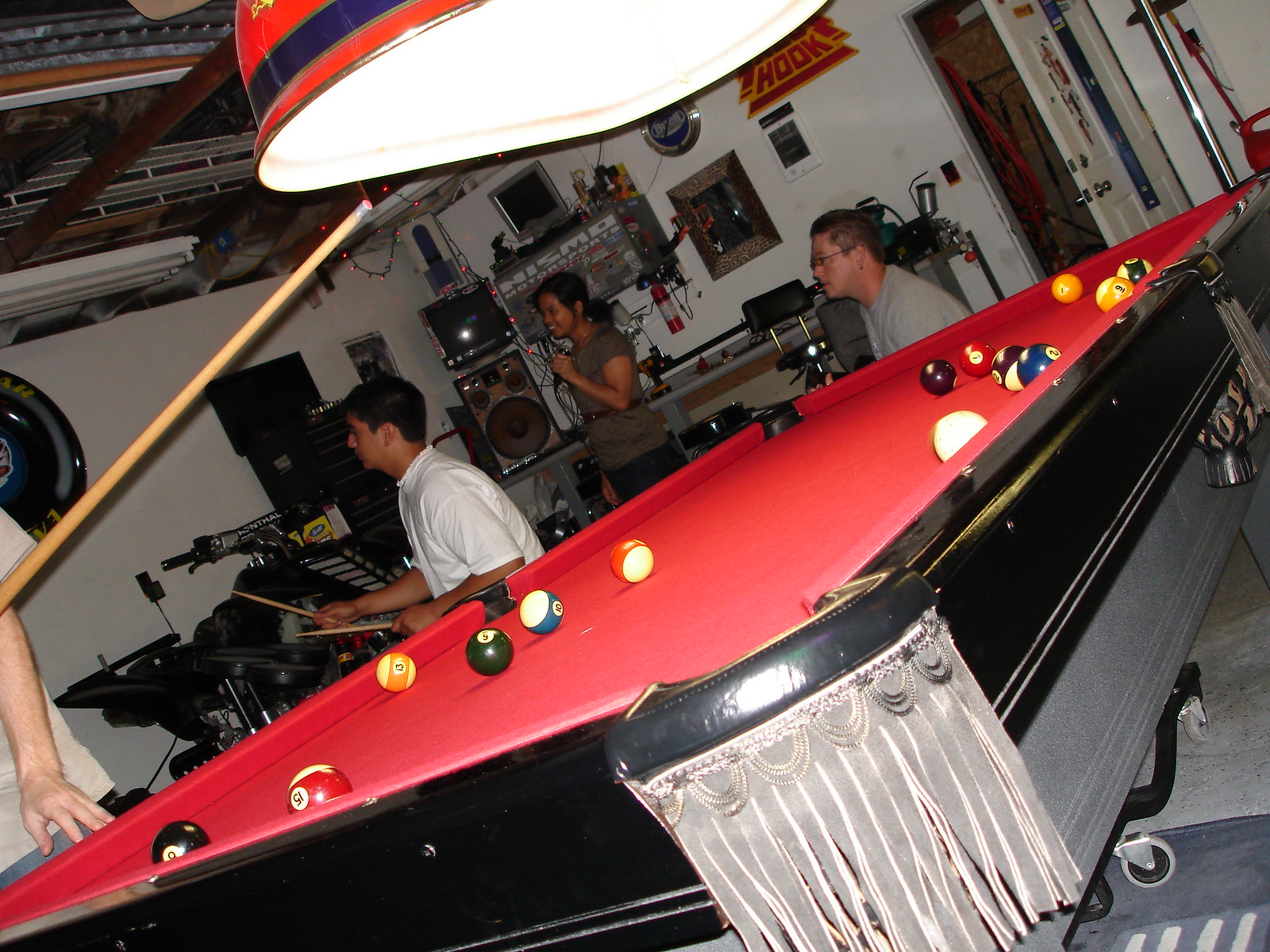In this cozy, possibly home-based or small-bar setting, the photograph captures a lively scene with various activities on display. The image prominently features a pool table with vibrant red felt, surrounded by a black and gray base, and pockets decorated with fringe. Scattered billiard balls suggest an ongoing game, with a person holding a pool cue entering the frame from the bottom left. Overhead, festive Christmas lights and a red hanging lamp trimmed in blue add a warm, colorful glow to the room.

In the background, a drummer, dressed in a white button-up shirt and seated at an electronic drum set, faces left as he plays. To his side, a woman in a brown short-sleeve top sings into a microphone, embracing the karaoke ambiance. Further back to the right, a man in glasses and a gray shirt sits, observing the scene. The room's unfinished ceiling with visible metal beams, UV lights, and white walls suggest a casual, perhaps makeshift entertainment space. Behind the performers, multiple speakers and electronic equipment, along with an open door revealing storage items like mops or rakes, complete the eclectic and vibrant setting.